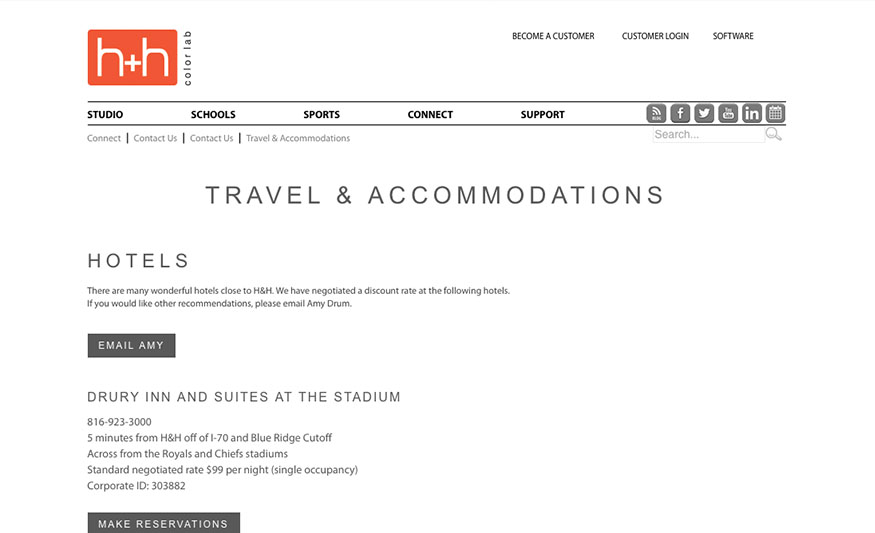**Detailed Caption:**

The image showcases a screenshot of a webpage from H+H Color Lab. The logo, prominently displayed at the top, features a red rectangle encasing two lowercase 'h's with a plus sign situated between them. In the upper right section of the page, there are three main navigational links: "Become a Customer," "Customer Login," and "Software," which are aligned horizontally and separated by thin black lines for clear distinction.

Below these menu options, another set of navigation tabs is present, offering categories such as "Studio," "School," "Sports," "Connect," and "Support." The navigation bar is adorned with social media icons, including those for Facebook, Twitter, LinkedIn, and an RSS feed.

The page currently displayed is the "Travel and Accommodations" section. This section provides detailed information about nearby hotels that offer discounted rates for those visiting H+H Color Lab. The text explains that several excellent hotels are in close proximity to H+H, with negotiated rates for their guests. 

One highlighted option is the "Three n Suites at the Stadium," located five minutes away from H+H near I-70 and Blue Ridge Cutoff, across from the Rails and Chiefs Stadiums. The hotel offers a standard negotiated rate of $99 per night for single occupancy. The Corporate ID for making reservations is 303882. For more assistance or inquiries, visitors are encouraged to email Amy Drome, with a conveniently placed button labeled "Email Amy" provided in black and white.

The navigation bar also includes additional options like "Connect" and "Contact Us," listed twice for emphasis, as well as "Travel and Accommodations," although these aren't detailed in the visible screenshot.

Overall, the page appears to be part of an art-related school or professional establishment, given the context of travel arrangements for students or visiting customers.